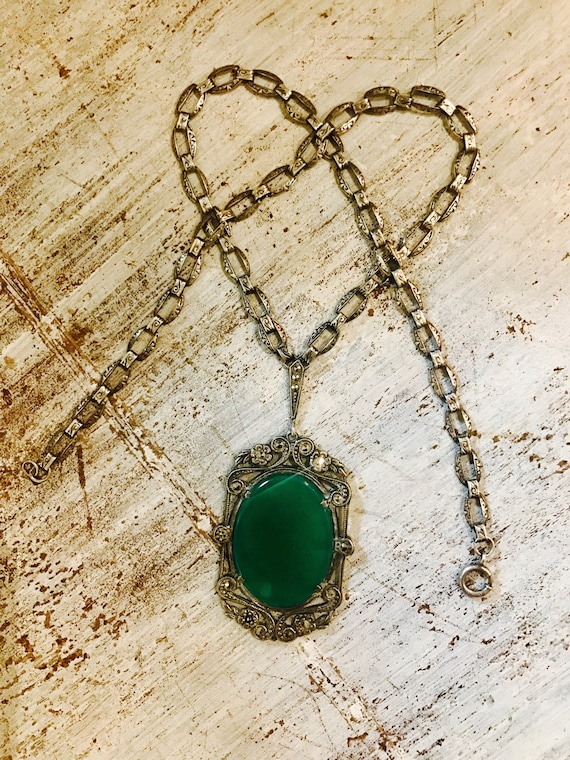The image depicts an elegant necklace artfully arranged on a weathered wooden surface, showing intricate details of both the jewelry and its backdrop. The necklace features a radiant green oval-shaped stone, possibly an emerald, encased in an ornate gold setting. The gold chain is quite robust and is meticulously laid out in a heart shape, emphasizing the visual appeal. The surface beneath has a tan hue with various stains and scratches, suggesting extensive use and adding character to the presentation. Light enters from the right, casting subtle shadows and highlighting the necklace's glossy and intricate details, transforming the display into a piece of art.